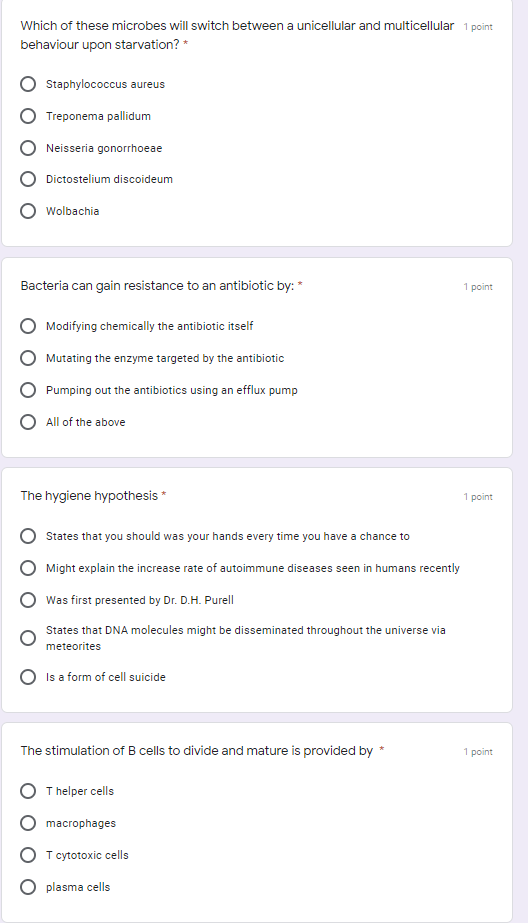The image depicts four distinct test questions arranged in a vertical stack against a white background. The text is black. 

1. The first question asks: "Which of these microbes will switch between unicellular and multicellular behavior upon starvation?" The options provided are: Staphylococcus aureus, Treponema pallidum, Neisseria gonorrhoeae, Dictyostelium discoideum, or Wolbachia. This question is worth one point.

2. The second question inquires: "Bacteria can gain resistance to an antibiotic by which of the following methods?" The possible answers are: modifying chemically the antibiotic itself, mutating the enzyme targeted by the antibiotic, pumping out the antibiotics using an efflux pump, or all of the above. This question is also worth one point.

3. The third question explores the hygiene hypothesis, providing various statements to choose from: "The hygiene hypothesis states that you should wash your hands every time you have a chance," "might explain the increased rate of autoimmune diseases seen in humans recently," "was first presented by Dr. DH Purell," "states that DNA molecules might be disseminated throughout the universe via meteorites," or "is a form of cell suicide."

4. The fourth and final question asks: "The stimulation of B cells to divide and mature is provided by which of the following?" The options are: T helper cells, macrophages, T cytotoxic cells, or plasma cells.

Each question is clearly delineated, offering a straightforward format for responding to the inquiries presented.